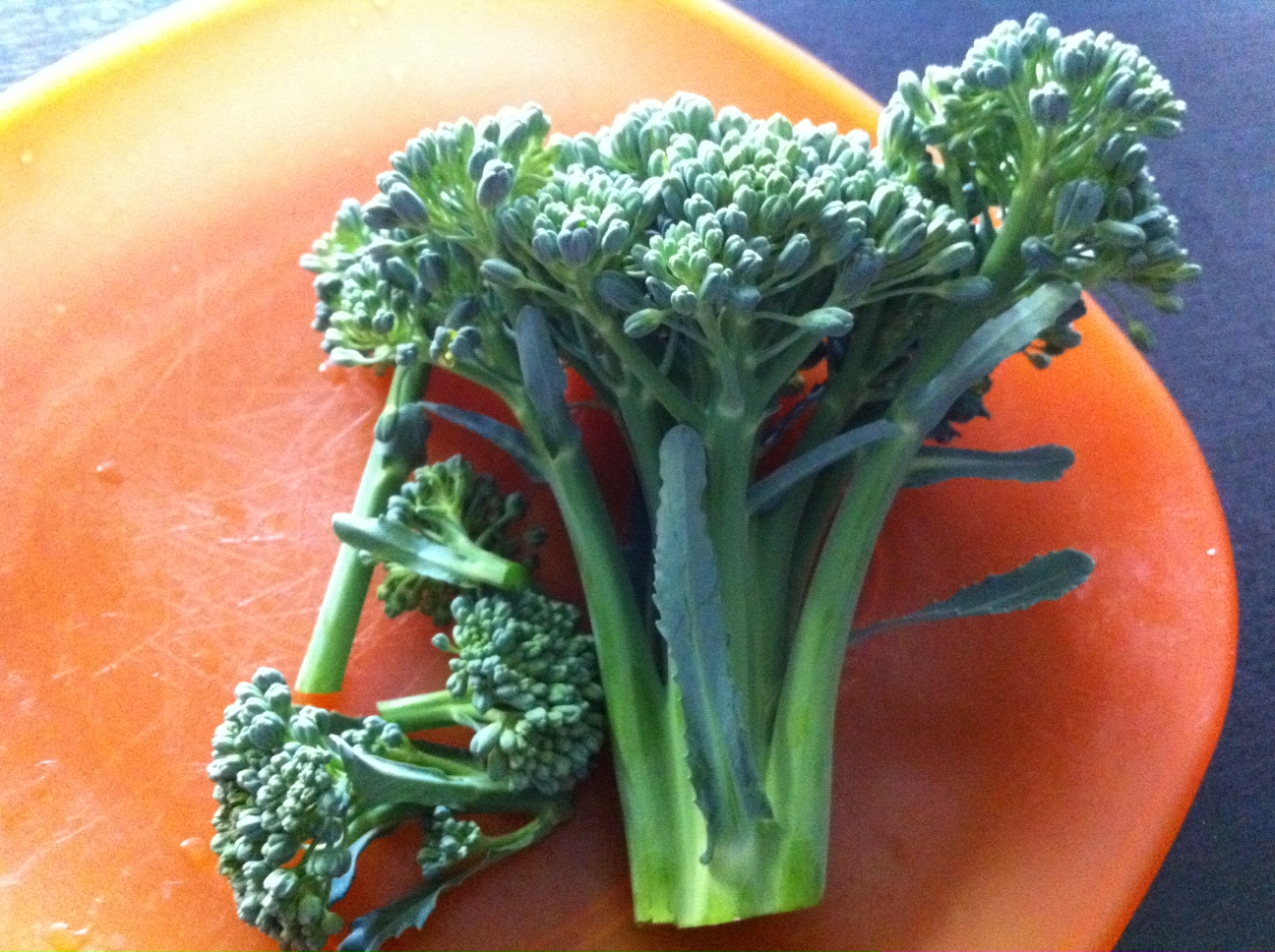This close-up image features an orange plate with a yellowish tint, showing evident signs of wear with several scratches. On the plate, which rests on a blue surface, sit pieces of broccoli. The largest piece, positioned upside down and a bit left of the center, is a whole stalk with some leaves attached. Surrounding it are several smaller broccoli florets, appearing somewhat scattered. The broccoli has a slightly dry appearance, with remnants of water droplets suggesting it was recently washed. Some parts of the broccoli exhibit a pale white film, and a section looks a little blue, prompting questions about its freshness. The lighting emphasizes the textures of both the plate and the broccoli, capturing every detail, from the smallest floret to the gray-green leaves.